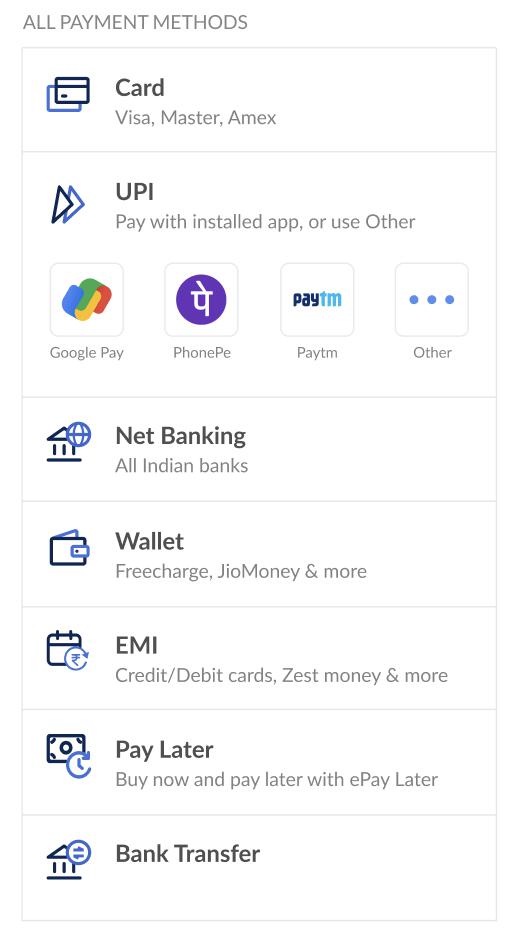This image displays a comprehensive "All Payments Method" screen. At the top, there's a section dedicated to card payments, listing Visa, MasterCard, and Amex cards. Following this, the screen offers several alternative payment methods: 

- **UPI**: Users can select this option to pay through the Unified Payments Interface.
- **Pay with Installed App**: This allows payment via apps already installed on the user's device.
- **Other**: An expandable option, represented by three dots, indicating the availability of additional choices.

Further down, several specific payment platforms are listed:

- **Google Pay**
- **PhonePe**
- **Paytm**
- **Other Options**: Again indicated with three dots for additional selections.

The image then outlines other categories of payment methods:

- **Net Banking**: Lists all Indian banks.
- **Wallet Payments**: Includes options like FreeCharge, Jio Money, and more.
- **EMI (Equated Monthly Installments)**: Offers payment through Credit or Debit Cards, ZestMoney, and other schemes.
- **Pay Later**: Describes a "Buy Now, Pay Later" option via ePayLater.
- **Bank Transfer**: Allows direct bank transfers as a payment method.

Each payment type is clearly categorized, giving users a wide array of choices for completing their transactions.